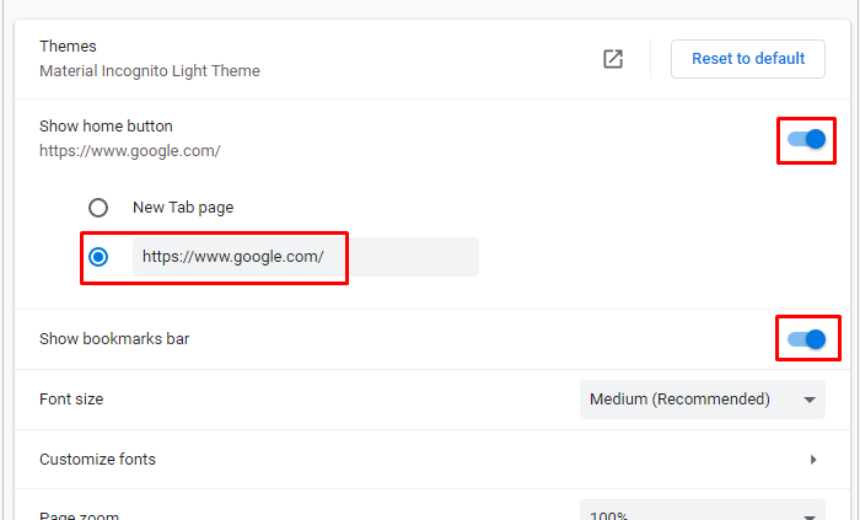The screenshot features a settings page with a light grey background and a prominently displayed white rectangular section with subtly rounded corners. This main area is divided into horizontal segments by thin grey lines for better organization. 

In the first section labeled "Themes," there are multiple options listed, including "Material," "Incognito," and "Light Theme." On the far right, a light grey box featuring an upward and rightward pointing arrow is present. Below this section, a button outlined in thin grey and filled with blue text that reads "Reset to Default" separates the themes section by another thin grey line.

Proceeding to the second section, it states "Show home button" followed by a URL: "https://www.google.com/." This area includes two radio buttons with grey outlines: the first, labeled "New Tab Page," is unselected and filled with white; the second, associated with "https://www.google.com/" in a light grey box, is selected with a blue fill and outline. Notably, this option is highlighted with a red outline, radio button included. At the top right of this section, a selection button (toggle or checkbox) is highlighted and selected.

The subsequent segment features a blue circle on the right and a light blue pill shape on the left, all enclosed in a red outline. Following this, another section discusses the "Show bookmarks bar" option, featuring an identical selection button also highlighted in red.

The final section addresses "Font Size" with a grey drop-down box that displays "Medium" accompanied by the word "Recommended" in parentheses. A grey arrow points downward to the right, indicating more options available within the drop-down.